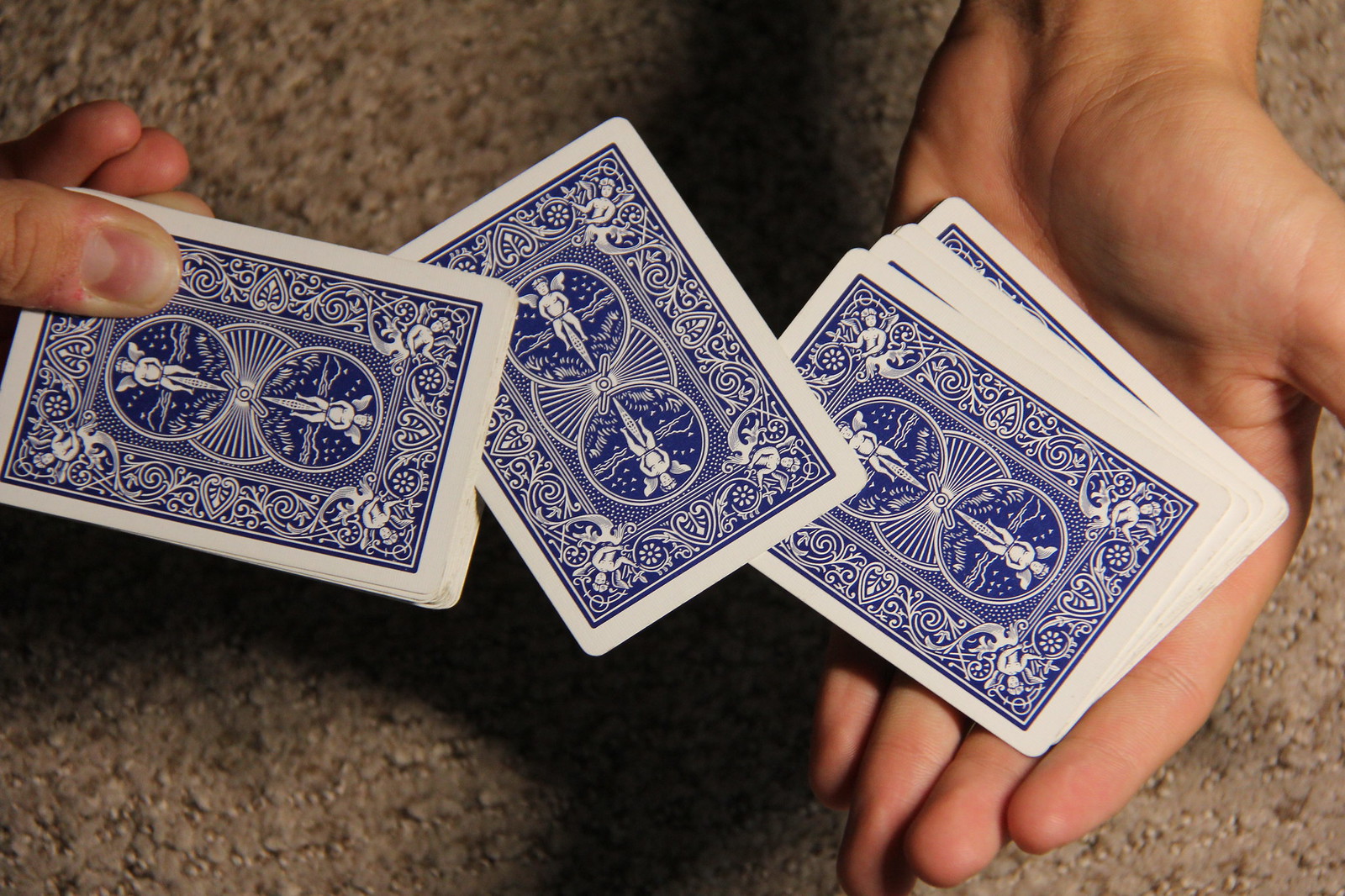In this detailed photograph, the background features a pristine beige shag carpet, indicative of a newer, unworn look. The focal point of the image is a pair of hands delicately holding a deck of playing cards. The left hand is prominently displayed, showing the palm fully open. On the right side of the image, the thumb and several fingers of the right hand are visible as well. 

The hands are handling what appears to be a complete deck of playing cards, although only six cards are clearly visible. The cards are shown from the back, revealing an intricate design rather than any suits or numbers. The card backs are primarily white, adorned with an elaborate royal blue design. This design is rich with filigree and features two central circles, each containing stylized images resembling fairies or angels, surrounded by intricate vines and hearts. A white border frames each card, adding to their ornate appearance.

Specifically, the thumb and fingers of the left hand hold a single card. The palm supports four cards, fanned out for better visibility of their detailed backs. Between these two groupings, another card is balanced and angled carefully, creating an aesthetically pleasing arrangement.